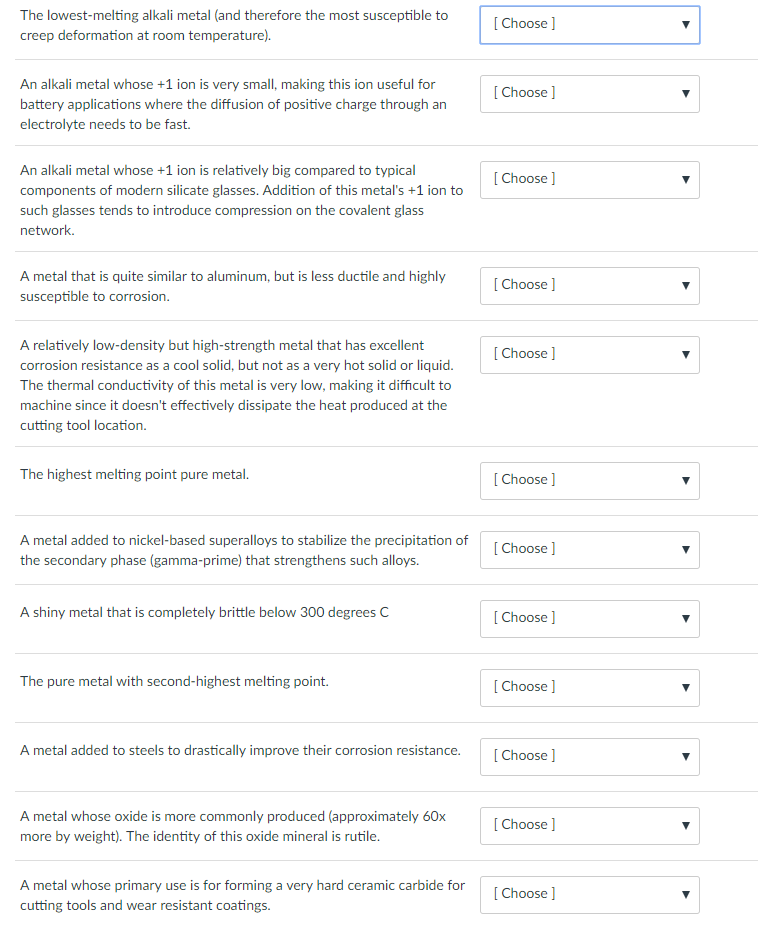This image is a screenshot of a chemistry quiz featuring multiple-choice questions arranged vertically. Each question has a drop-down menu for selecting the correct answer. 

- The first question asks for the identity of the lowest melting alkali metal, which is also the most susceptible to deformation at room temperature.
- The second question seeks the name of an alkali metal with a very small +1 ion, making it ideal for battery applications due to its fast diffusion of positive charge through an electrolyte.
- The third question inquires about an alkali metal whose relatively large +1 ions introduce compression to the glass network when added to modern silicate glasses.
- The next question is about a metal that resembles aluminum but is less ductile and highly prone to corrosion.
- Another question describes a metal with low density but high strength, known for its excellent corrosion resistance in its solid state, though this resistance diminishes when it is very hot or liquid. This metal also has poor thermal conductivity which poses machining challenges.
- There is a question about the metal with the highest melting point.
- Another question asks for the metal added to nickel-based superalloys to stabilize the precipitation of the secondary phase gamma prime, which strengthens these alloys.
- One question describes a shiny metal that becomes completely brittle below 300 degrees Celsius.
- Next, the quiz asks for the metal with the second highest melting point.
- Another question seeks the metal added to steels to significantly enhance their corrosion resistance.
- One question identifies the metal whose oxide is predominantly produced, with rutile being the most common form of this oxide mineral.
- Lastly, the quiz asks for the metal primarily used in forming a very hard ceramic carbide for cutting tools and wear-resistant coatings.

This detailed summary highlights the nature of the questions within the chemistry quiz, focusing on various metals and their unique properties and applications.